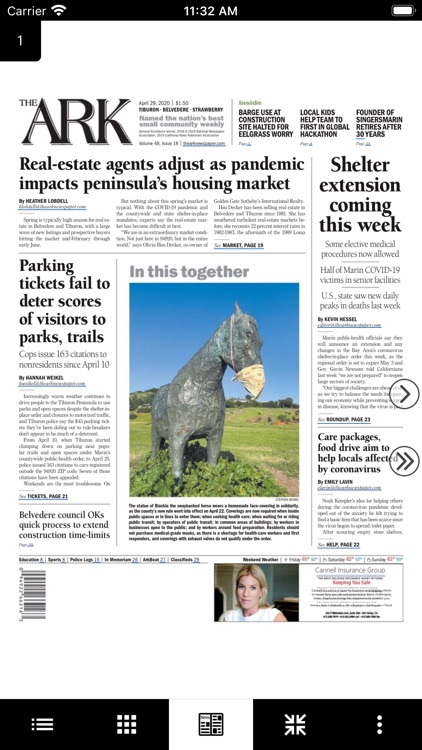A detailed caption of this image could be:

"A mobile phone screen displays a newspaper article from 'The Arc' publication. The article, titled 'Real Estate Agents Adjust as Pandemic Impacts Peninsula's Housing Market,' features a central image of an aged, oxidized metal statue of a horse wearing a white mask. The statue stands against a backdrop of green grass and a blue sky. Additional visible headlines include 'Shelter Extension Coming This Week' and 'Parking Tickets Failed to Deter Scores of Visitors to Park Trails.' The background of the newspaper is predominantly white with black text, emphasizing the contrast and clarity of the content on the mobile device."